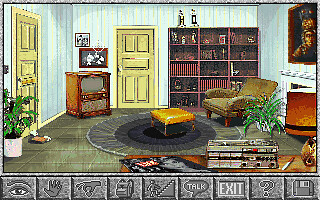This image is a horizontal rectangular screenshot of an old computer video game, reminiscent of the 80s or 90s with very basic and pixelated graphics that could be 16-bit or 64-bit. The scene is depicted from a first-person perspective and portrays the interior of a den or living room. The room features blue or white-paneled walls and a beige-green floor. Prominently, there are two yellow doors, one on the front and another possibly on the left-side wall. A gray-green or green recliner chair sits just off to the right, complemented by a yellow ottoman in the center.

Along the back wall, there's a brown wooden bookshelf filled with books and curios. On the right side of the room, a gray-green chair resides near a fireplace with a red and orange fire lit, above which hangs a large photograph or painting. In the left corner flaunts an old-fashioned console TV set. Additional furniture includes a table with a black carpet underneath, which holds a radio, a cigarette, and a magazine.

Along the bottom of the image, a gray bar spans horizontally, showcasing various interactive icons: an eye, a hand, a hand grasping some money, a backpack, a figure ascending stairs, a speech bubble labeled "talk," an "exit" sign, a question mark, and a diskette symbol for saving progress. These icons suggest different commands or actions the player can perform within the game.